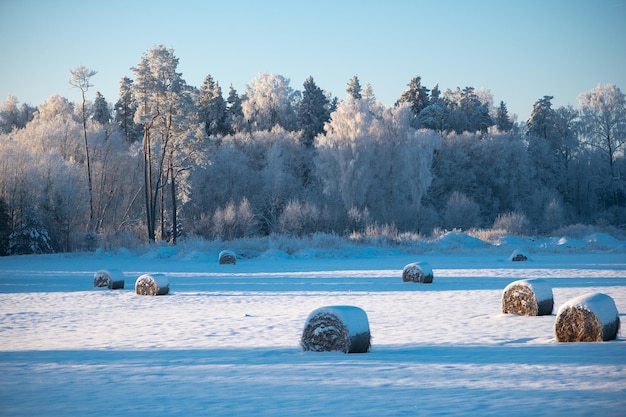This is a picturesque winter scene of a snowy farm field. In the foreground, seven large bales of hay, partially covered in snow, stand in a vast blanket of white that stretches across the entire area. The ground is fully enveloped in heavy snow, creating a serene, uninterrupted landscape. In the background, a dense forest stands tall, with trees cloaked in a mixture of green foliage and thick, white snow, giving a stark, beautiful contrast. Smaller shrubs and plants can be seen dotting the area beneath the trees, their colors muted by the snow. The sky above is a clear, bluish-gray without any clouds, framing the peaceful winter scene. The combination of the snow-laden trees, the blanketed field, and the hay bales, with bits of snow settled on top and on the sides, creates a tranquil and cohesive winter panorama.